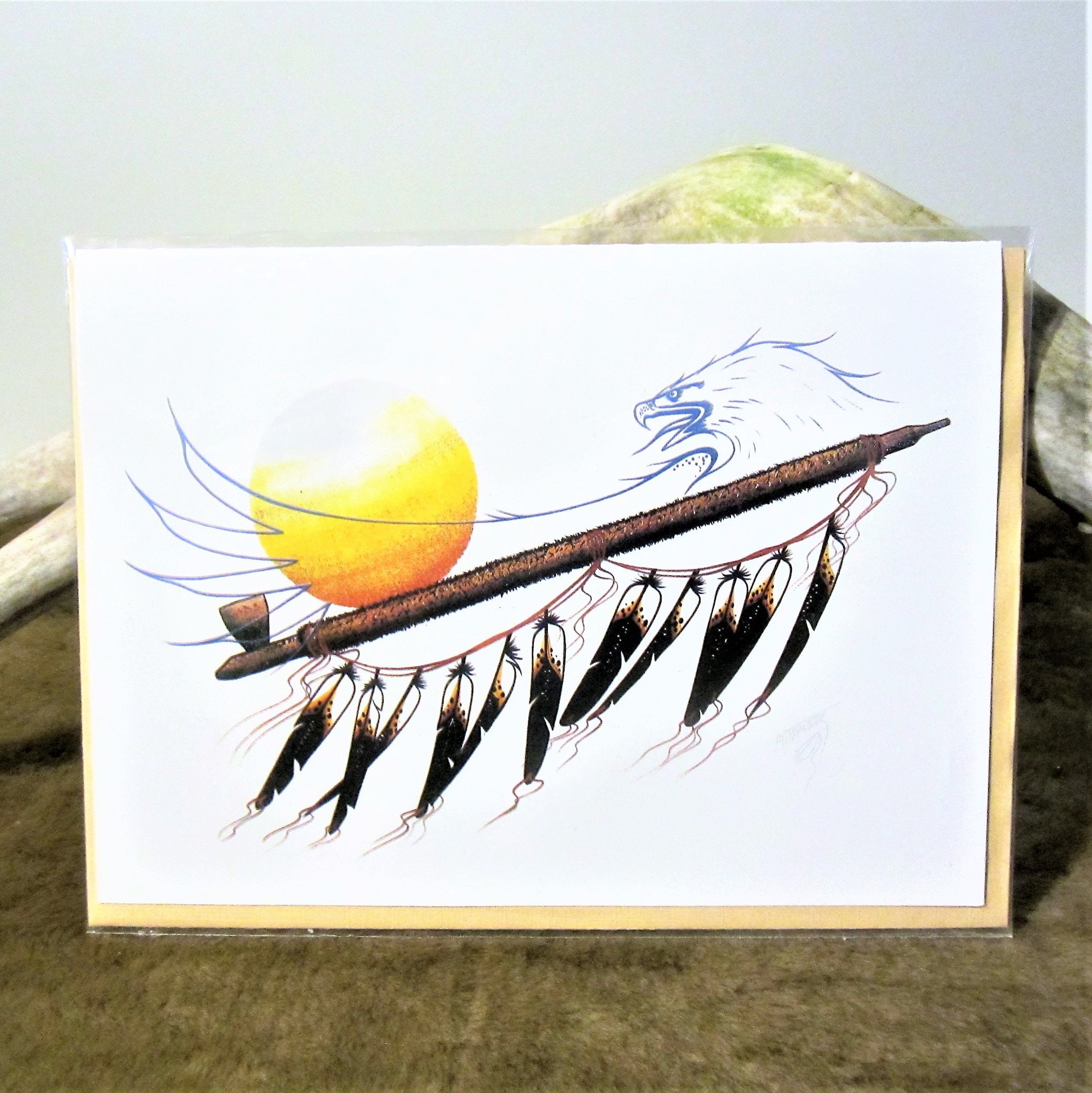The image is a square color illustration that appears to be photographed. The illustration is displayed on a large poster board encased in a clear plastic sleeve for protection. This poster board is propped up against a piece of wood and placed on a textured, carpet-like flooring. 

The illustration itself depicts a traditional Native American peace pipe adorned with feathers, which hang from strings tied to the pipe. Above the peace pipe, there is a detailed drawing of an eagle, which may be a representation of a golden or bald eagle, with its beak open as if in mid-call. The eagle's head, along with one wing, is clearly visible and watching towards a sun, colored with sunset hues of yellow and orange. The background of the photograph is somewhat ambiguous, featuring a beige carton-like surface with a 3D appearance and shades of green and grey, possibly representing a natural setting. The overall composition of the image combines cultural symbolism with detailed artistry, capturing the viewer's attention through its vivid depiction of Native American elements and the majestic eagle.